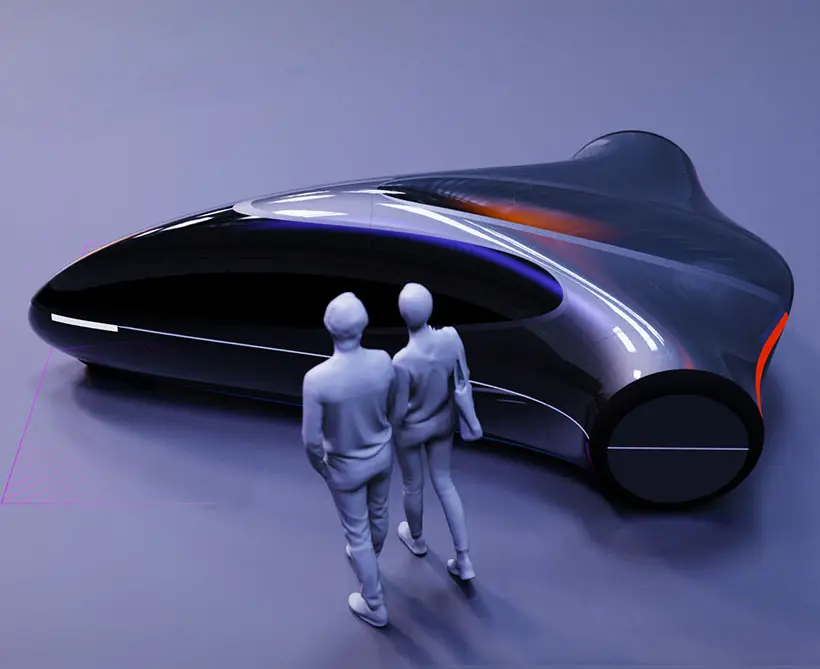In this digitally rendered image, a sleek, futuristic vehicle takes center stage, evoking the aesthetic of a spacecraft adapted for terrestrial travel. The vehicle, with its pointed front and bulbous rear, is crafted from a smooth, silver metallic material and features a large, tinted black window that wraps around the front. Two prominent rear wheels are visible, accentuated with striking red taillights, adding a dynamic touch to its avant-garde design.

Situated against a gradient background that transitions from light bluish-purple to gray, the scene is detailed with careful shadowing from the vehicle, enhancing its three-dimensional presence. In the foreground, two unpainted, gray figurines represent a man and a woman walking towards the vehicle. The man, dressed in a long-sleeved shirt and pants with sneakers, and the woman, identifiable by her purse slung over her right shoulder and her sneakers, are depicted in a minimalist, clay-like style, with smooth contours and devoid of facial features.

The flooring beneath them appears paper-like in texture, blending into the overall soft and futuristic ambiance of the image. The meticulous details—including the red reflections on the vehicle and the textural nuances of the models—combine to create a vivid and immersive depiction of a scene straight out of a sci-fi realm.